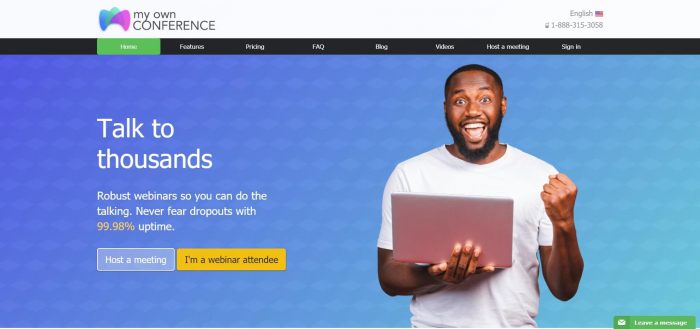This screenshot captures the home page of the "My Own Conference" website. In the top left corner, the "My Own Conference" logo features colorful abstract shapes. A navigation bar spans the top, offering the following options: Home, Features, Pricing, FAQ, Blog, Videos, Host a Meeting, and Sign In. To the right of the navigation bar, language selection and contact information, including a phone number, are available.

The background of the page transitions from light blue to dark blue, adorned with a subtle pattern of dots and circles. Prominent text reads "Talk to thousands" followed by smaller text that advertises "Robust webinars so you can do the talking. Never fear dropouts with 99.98% uptime." Below these messages, there are two buttons: a blue one labeled "Host a Meeting" and a yellow one labeled "I'm a Webinar Attendee."

On the right side of the page, there is an image of a smiling man holding a laptop with a surprised expression, as if saying, "Alright!" In the bottom right corner of the page, a green button labeled "Leave a message" is visible. The layout and design elements effectively highlight the platform's features and encourage user interaction.